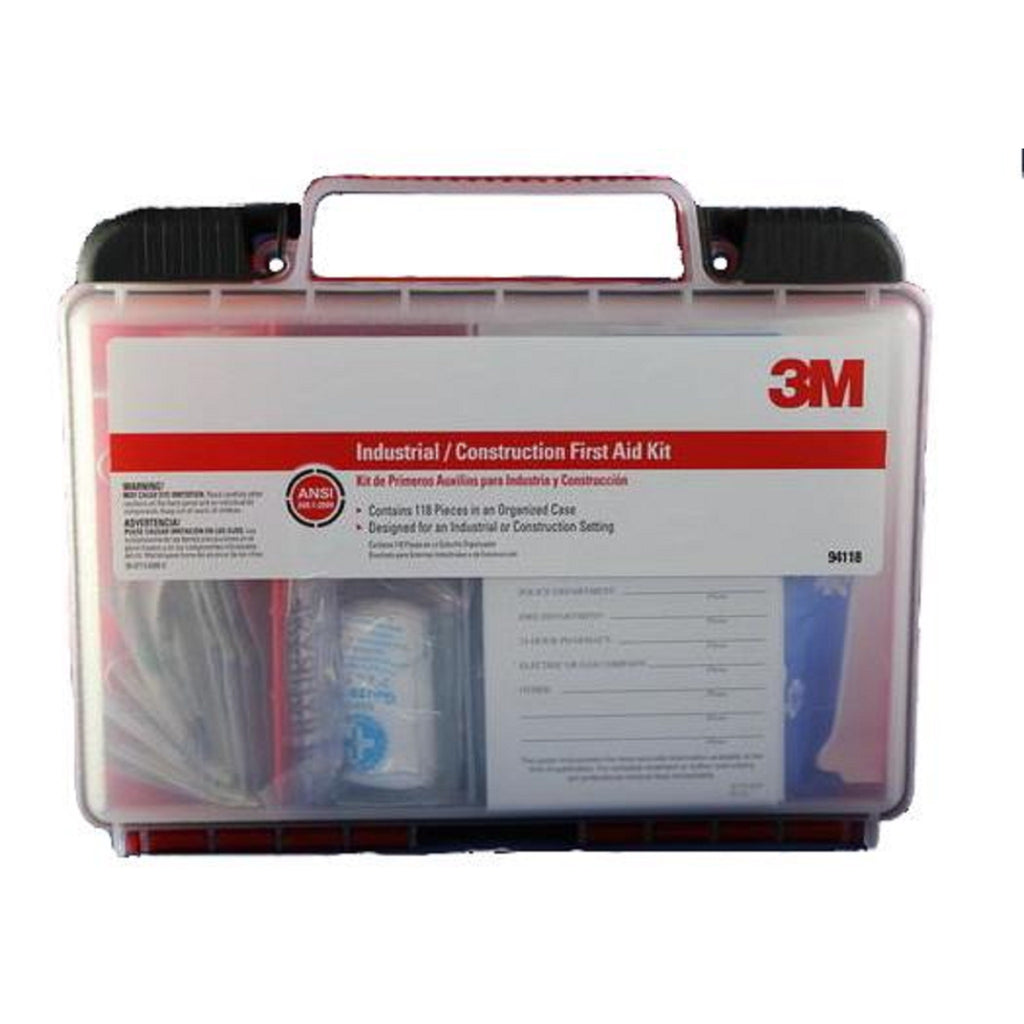This is an image of a square, transparent industrial construction first aid kit branded by 3M. The case, which has a slightly opaque, white-tinted lid made from injection-molded plastic, is standing upright and facing the camera. At the top, it features a carrying handle and two black clips that keep the kit securely shut. The front of the kit has a label with a red bar across it, displaying essential information including the brand logo (3M), and mentions that it is ANSI approved. The label states that the kit contains 118 pieces and is specifically designed for construction settings. There are various warning labels and text in multiple languages, with a reference number 94118 in the bottom right corner. Through the transparent lid, you can partially see some of the contents, including bandages, Band-Aids, a roll of gauze, and a sheet of paper that likely contains emergency contact information.